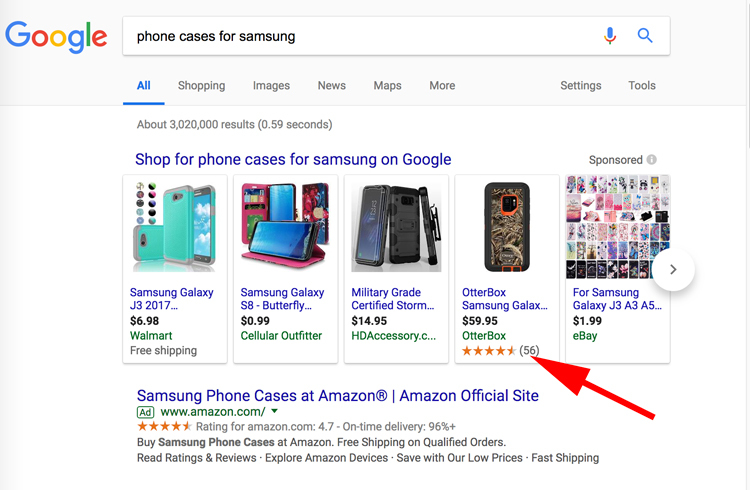This is a screenshot of a Google search results page for "phone cases for Samsung," displayed on an older device. The search bar is rectangular, a design characteristic from earlier interface models. To the left, the search query is displayed in black text. Below, the navigation tabs list options such as "All," "Shopping," "Images," "News," "Maps," and "More." All tabs are in gray except "All," which is highlighted in blue, bolded, and underlined. The page also shows a gray text line indicating it found about 3,020,000 results in 0.59 seconds.

Below this, a blue link invites users to "Shop for phone cases for Samsung on Google," followed by a showcase of different phone cases. The first image features an aquamarine case for the Samsung Galaxy J3 (2017). Multiple circular icons beneath this image indicate the availability of various colors and patterns. The price listed in bold black text is $61.98, and the seller is Walmart, providing free shipping as noted in green text below.

The second listing displays a pink floral case that doubles as a stand for the Samsung Galaxy S8. Its title has been truncated to "Samsung Galaxy S8 - Butterfly...". The price, in bold black text, is $0.99, sold by Cellular Outfitter, as indicated in green text.

The third case is a durable, military-grade certified, army-style design with a clip on the back. Its title, shown in blue, has been cut off with "Military Grade Certified Storm...". 

Overall, the search results provide a visually detailed collection of Samsung phone cases, each accompanied by descriptions, prices, and seller information.